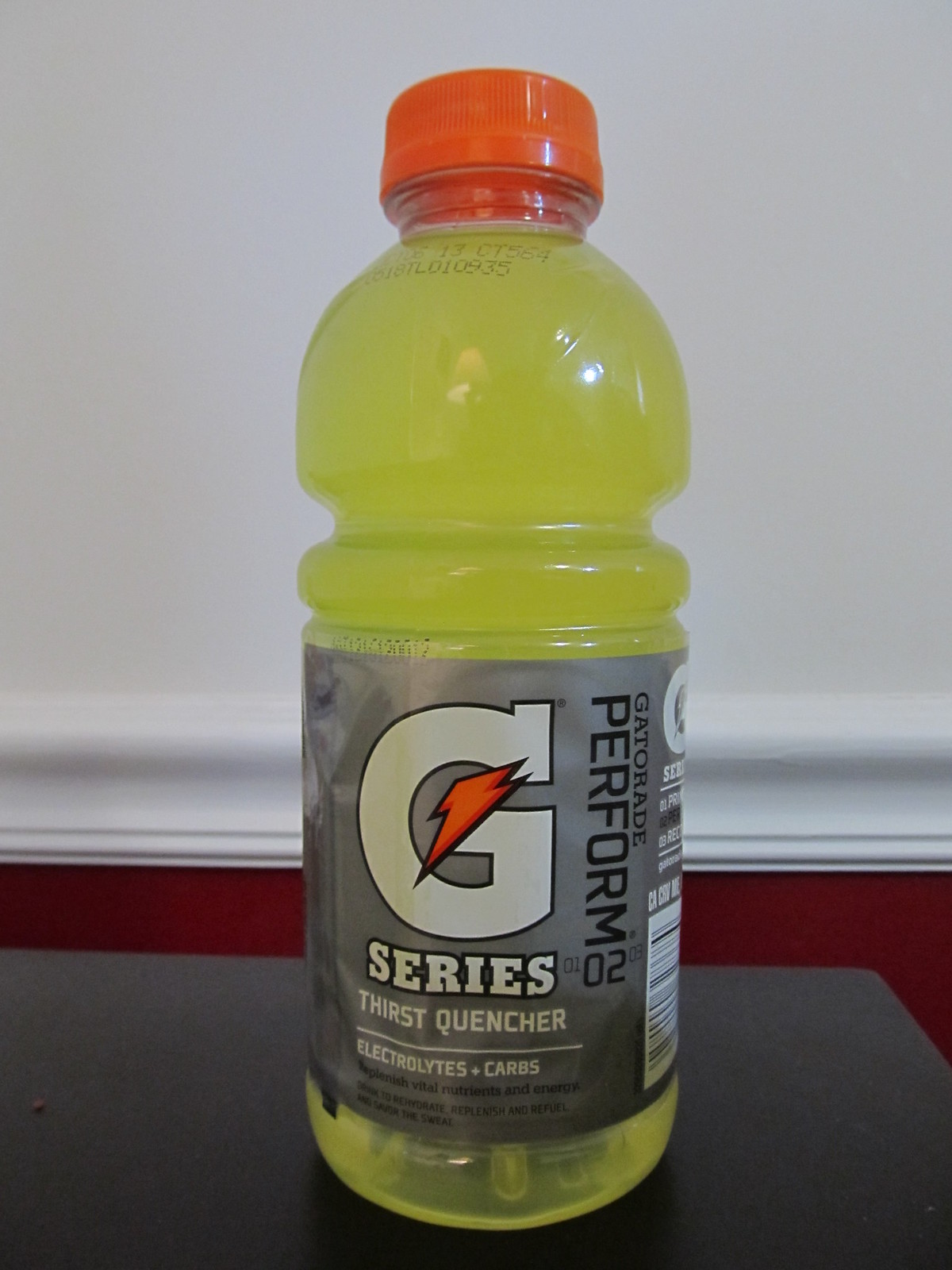A prominently displayed bottle of yellow Gatorade occupies the center of the image, positioned on a desk with a white wall serving as the backdrop. The clear, plastic bottle is part of the G-Series Thirst Quencher Perform 02 product line, known for its replenishing blend of electrolytes and carbohydrates. The detailed label, printed in gray, provides this nutritional information and stands out against the pale liquid inside. Topping the bottle is a bright orange cap, adding a pop of color. Around the neck of the bottle, printed numbers and codes are visible, likely for tracking and inventory purposes. This scene captures the familiar and ubiquitous sight of a Gatorade bottle, something instantly recognizable to many.